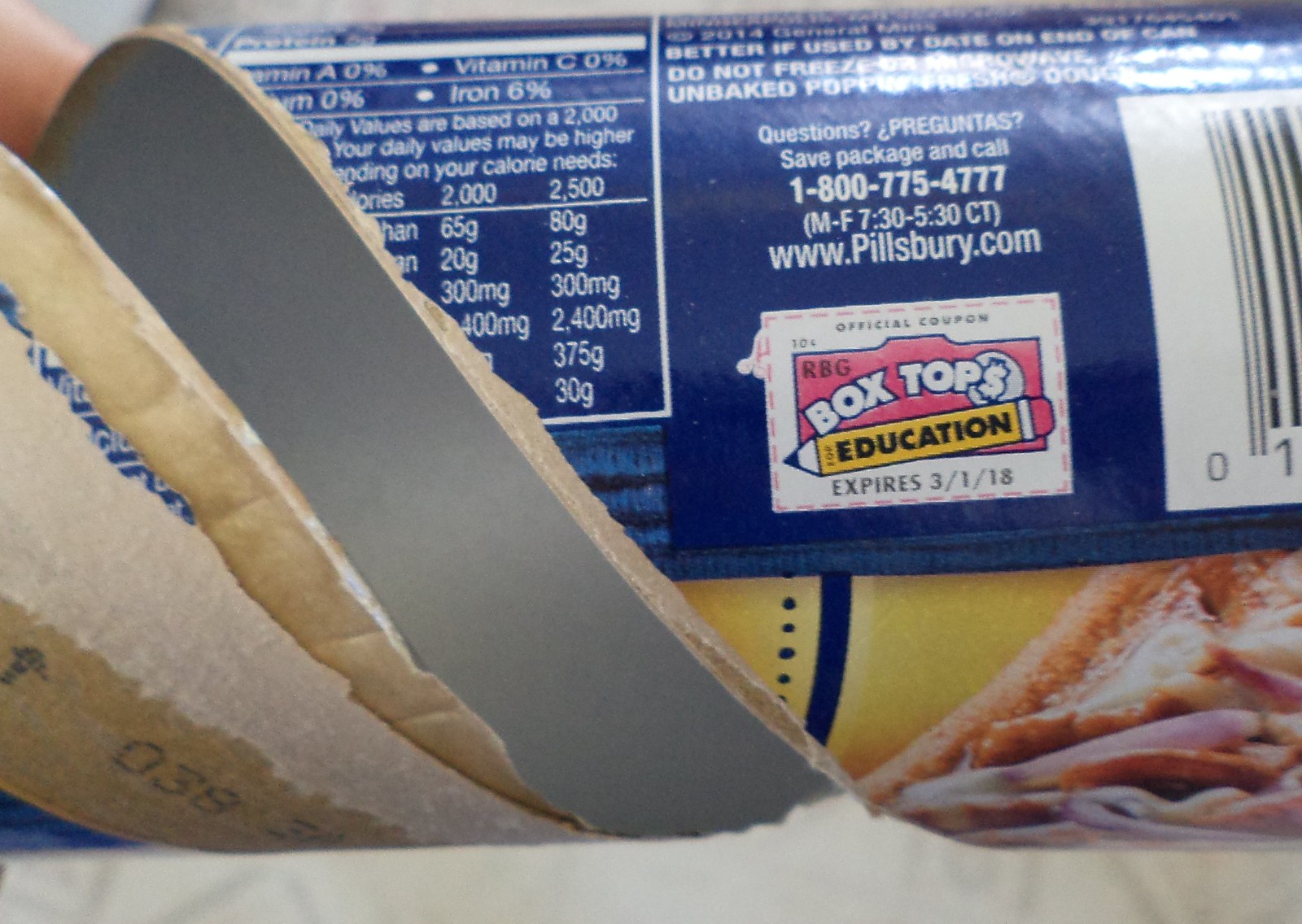The image depicts an unrolled Pillsbury canister, designed to hold bakery items such as instant bread, biscuits, or pastries. The cylindrical canister, constructed from a mix of paper and metal, prominently displays the Pillsbury logo along with the website URL, www.pillsbury.com. Essential details, including a toll-free customer service number, baking instructions, and some nutritional information, are visible on the wrapper. Additionally, a segment of the barcode and a "Box Tops for Education" label can be seen, indicating its contribution to school fundraising programs. This typical Pillsbury canister reflects the brand's dedication to quality and customer engagement.